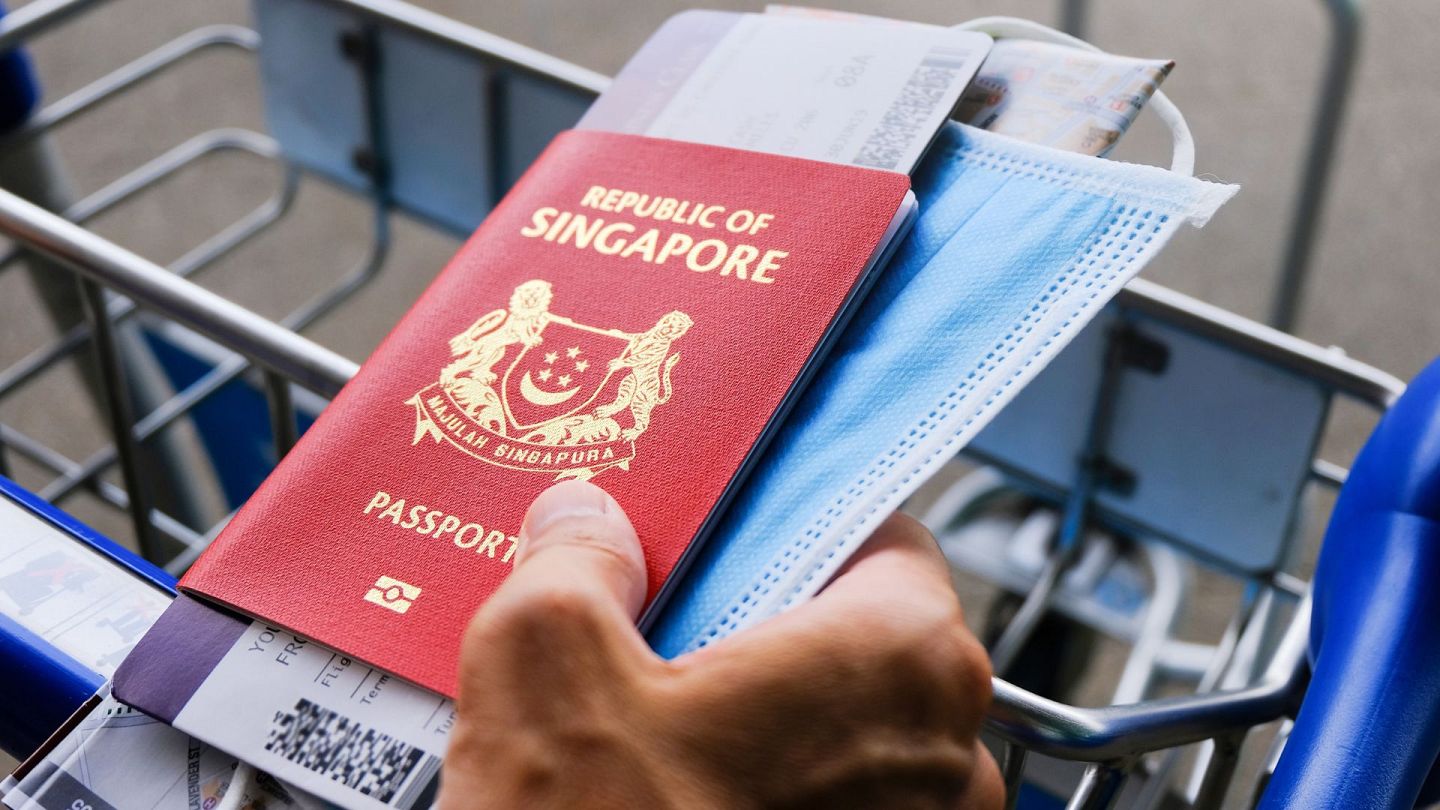In this detailed close-up color photograph, a tan-skinned right hand, slightly humid, is seen holding a collection of items over a metallic basket that appears to be part of a shopping cart or luggage trolley with silver framework and blue edges. The focal point of the photo is a red leather passport prominently featuring the gold-embossed text "Republic of Singapore" along with an insignia depicting a lion and a tiger flanking a shield with a crescent moon and five stars. Below the insignia, the word "passport" is also stamped in gold. Nestled beneath the passport are a partially visible purple-and-white flight ticket and a simple blue face mask with white borders. The background, slightly out of focus, suggests a metallic structure possibly for carrying luggage, clarifying the context of travel inherent in the image.